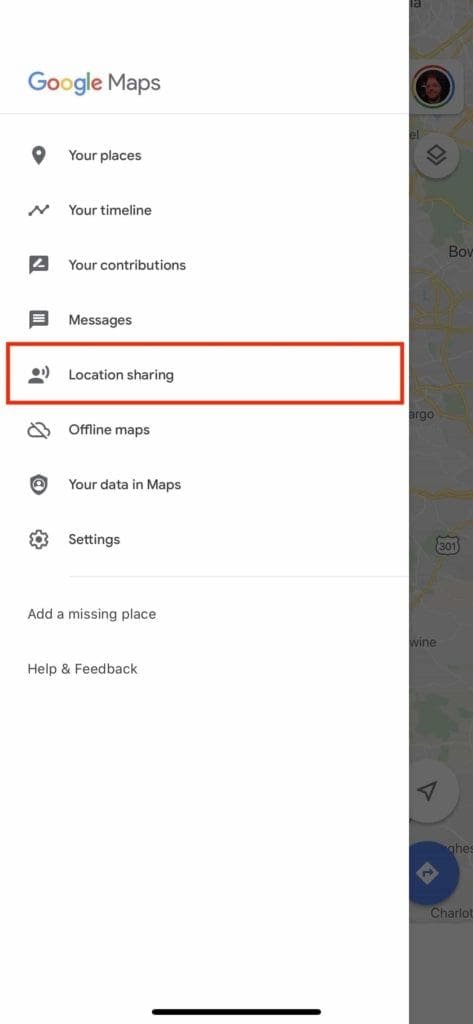This image is a screenshot from Google Maps, focusing on an expanded side menu. On the far right, a sliver of the actual map can be seen, although it is grayed out to emphasize the menu. The menu is a clean, white vertical bar located on the left side of the screen.

At the very top of the menu, the familiar Google Maps logo is featured, comprising the multi-colored Google logo with the word "Maps" adjacent to it. Directly beneath this logo is a subtle gray dividing line.

Following the divider, the menu items are listed as follows: 
1. An icon depicting a location pin next to the label "Your Places."
2. An icon of a bar graph labeled "Your Timeline."
3. An icon illustrating a pencil with the label "Your Contributions."
4. An icon of a speech bubble marked "Messages."
5. An icon showing a person with sound waves emanating from the mouth, labeled "Location Sharing" and circled in red to indicate active selection.
6. An icon of a cloud with a diagonal slash labeled "Offline Maps."
7. An icon resembling a shield with a human silhouette labeled "Your Data in Maps."
8. An icon of a gear, next to which is the label "Settings."

Finally, at the bottom of the menu, another gray dividing line precedes the options "Add a Missing Place," "Help," and "Feedback." This detailed layout underscores the various functionalities and personalization features offered within the Google Maps application.